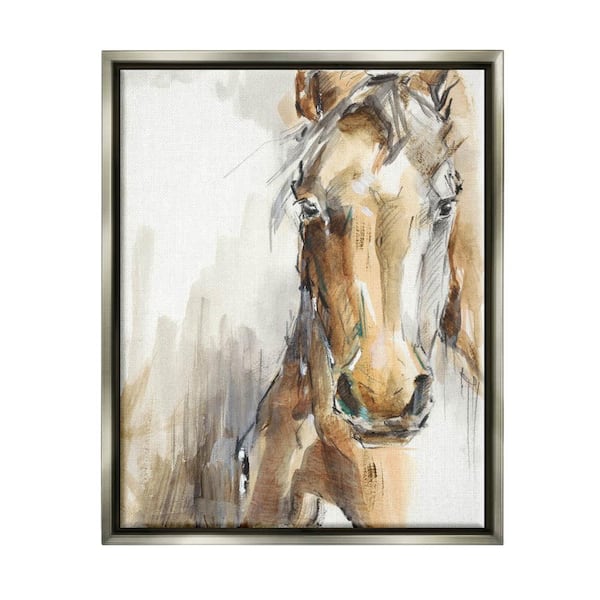The photograph captures a framed painting of a horse's head and neck, presented in a rectangular format with the longer sides vertically aligned. The frame itself is silver with an inner black border, surrounded by a large white border. The horse in the painting faces forward, its expressive eyes gazing directly at the viewer. Its head is intricately detailed, showcasing a blend of dark browns, light browns, and whites; the right side of its face is dark brown, transitioning to light brown in the center, and white on the left side extending to its neck. The background complements these earthy tones with strokes of black, gray, and brown, accented by a significant white spot in the top left corner. The painting, with its nuanced shading and lifelike depiction, brings the horse to life, focusing primarily on its elongated face and neck.